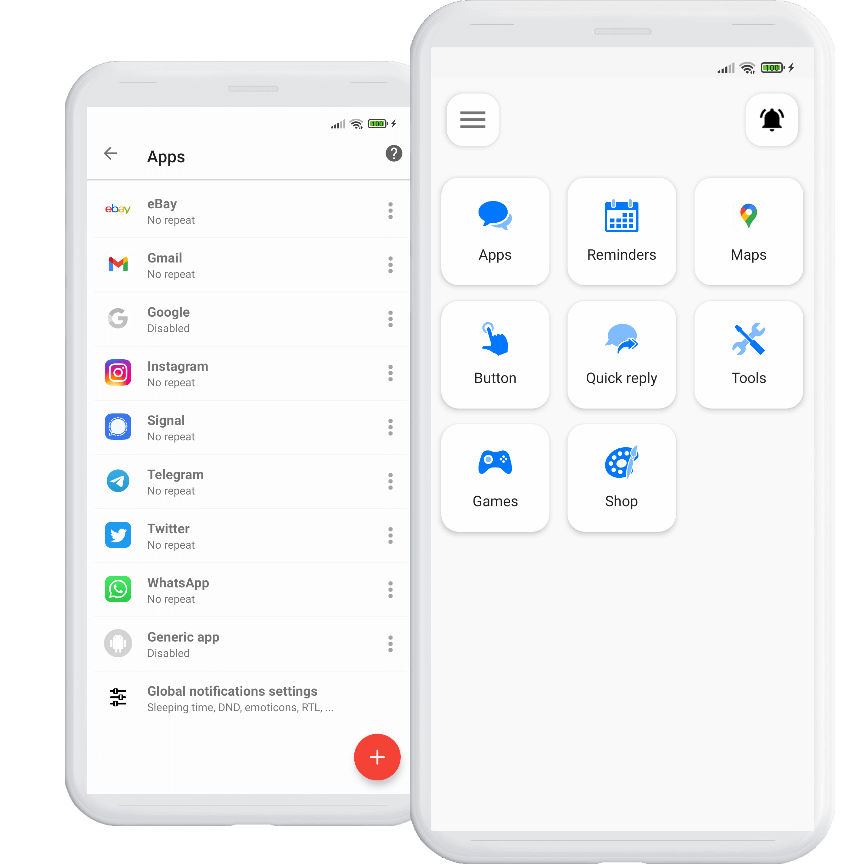The image features two white boxes on a white background. The first box is organized with a selection of app icons and has an arrow key pointing to the left. Adjacent to this, there is a question mark. Below these elements, there is a gray line with the following descriptions:

- "eBay" mentioned twice, indicating distinct entries but without repetition.
- Individual entries for "Gmail," "Google," "Instagram," "Signal," "Telegram," "Twitter," "WhatsApp," and "Generic App."
- "Global Notification settings," each paired with their respective icons.

At the bottom of this box, there is a distinctive red button featuring a plus sign.

The second box includes a speaker icon on one side and a ringing bell on the other. The top section displays the battery life indicator and Wi-Fi status. This box has multiple selectable buttons with various categories:

- "Apps," represented by a blue logo with the word "Apps" in black letters.
- "Reminders," symbolized by a blue calendar icon and labeled "Reminders" in black.
- "Maps," featuring the Google Maps symbol.

Additionally, there are buttons labeled:

- "Buttons" with an icon of a blue hand pressing a button.
- "Quick Reply."
- "Tools," represented by a blue screwdriver and wrench icon.
- "Games," illustrated with a game console icon.
- "Shop," accompanied by its corresponding symbol.

Overall, the image portrays a neatly arranged selection menu with various app and tool categories, each iconographically represented and labeled for easy identification.